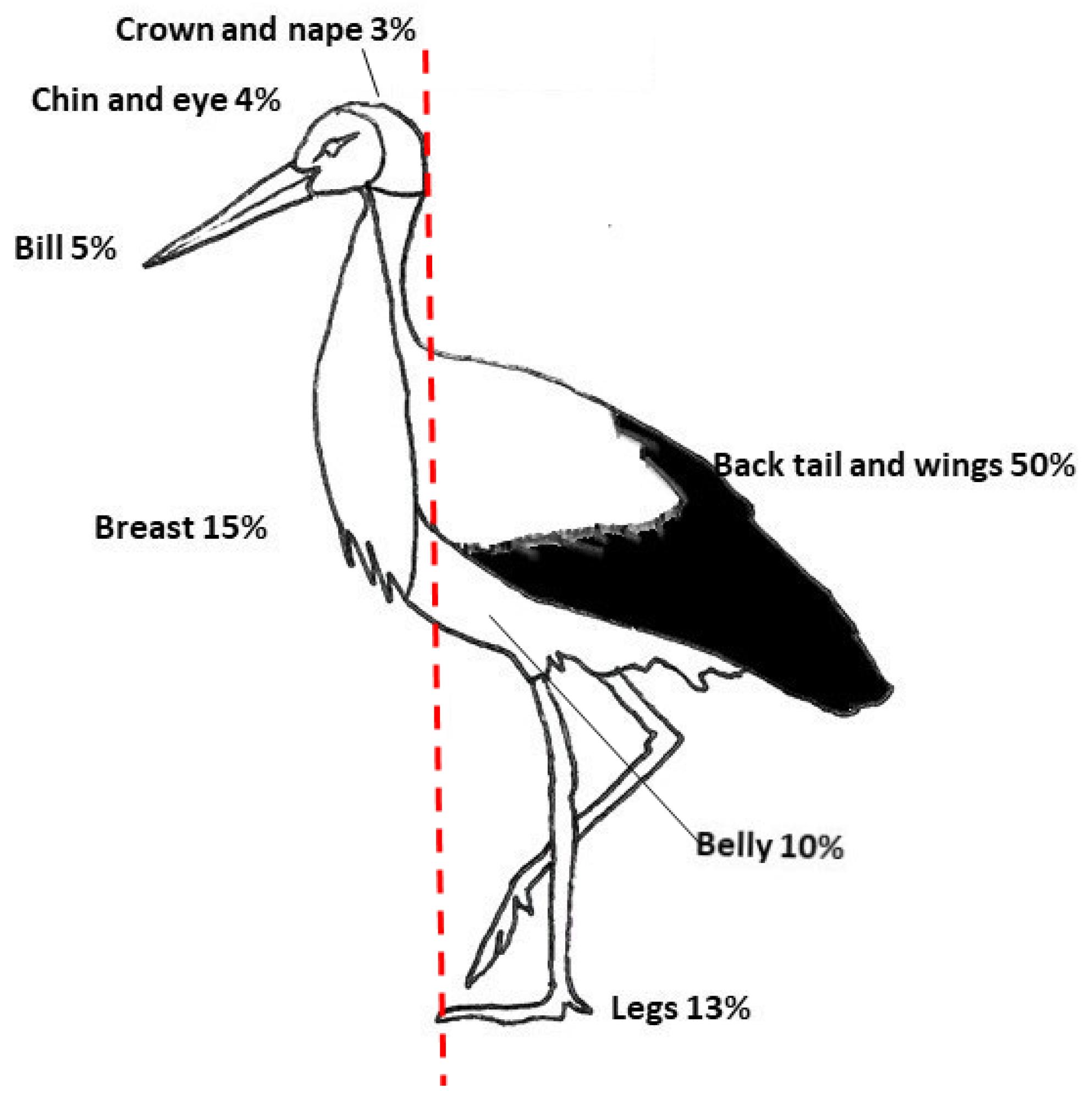The illustrated diagram features a sketched image of a stork, primarily black and white, with specific annotations. The bird, facing left, has black-tipped wings and stands with one leg lifted. A red dotted line vertically divides the image from the top of the head through the body, stopping in front of the feet. Black text denotes percentages likely representing the proportion of each body part within the image: "crown and nape, 3%," "chin and eye, 4%," "bill, 5%," "breast, 15%," "back, tail, and wings, 50%," "belly, 10%," and "legs, 13%." Notably, the label for "belly" includes a line pointing directly to the bird's underbelly, while other labels are adjacent to their corresponding parts without lines.